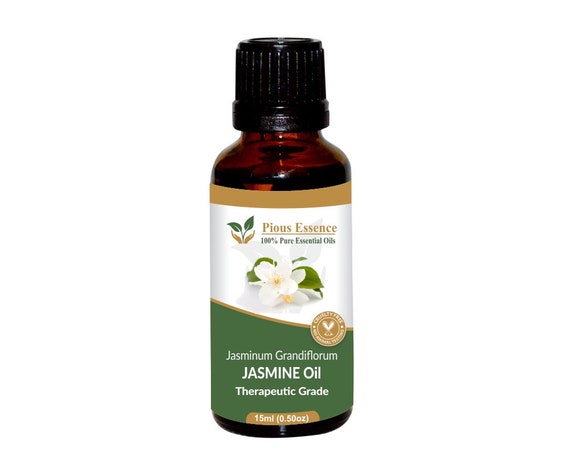This product image features a small, cylindrical brown glass bottle with a black cap set against a white background. The bottle is labeled with an olive green and white label that has a beige strip at the top. Prominently displayed on the label is the brand name "Pious Essence" followed by the text "100% Pure Essential Oils." Above this text is a logo depicting a hand holding leaves. Below the brand name, there is an image of a jasmine flower and leaves, and the text further specifies the product as "Jasminum Grandiflorum Jasmine Oil, Therapeutic Grade, 15 ml (0.50 OZ)." Additionally, the label features an emblem indicating that the product is "Cruelty Free." This essential oil bottle appears intended for use in aromatherapy and would likely be found on retail or health-focused websites.